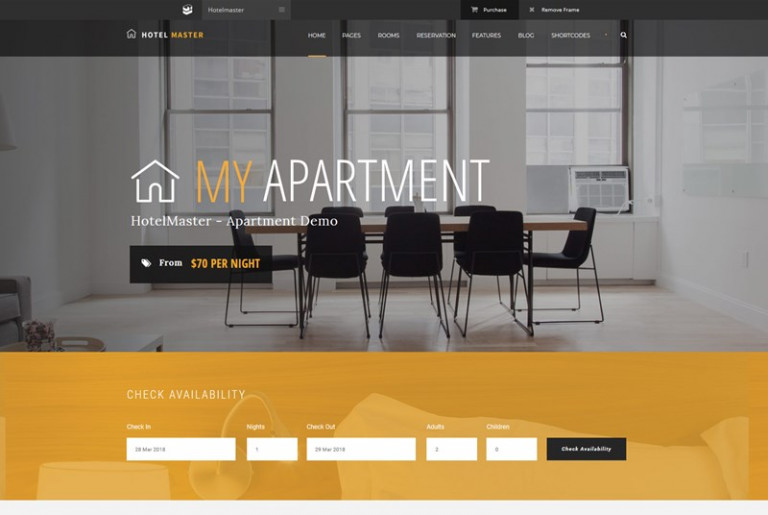The webpage features the "Hotel Master" website, prominently displayed with "Hotel" in white and "Master" in yellow on the top left corner of a black background. The header, which is also black, includes navigational tabs such as Home, Pages, Rooms Features, Blog, and Short Cooks, all written in white. Below the header, the background image showcases the interior of a house with a wooden office or conference desk surrounded by eight black chairs. The flooring is gray, and the surrounding walls are white. The room features three windows positioned in front of the chairs. Centrally located on the page, there is text stating "My Apartment Hotel Master Apartment Demo," accompanied by an image of a house taken by a drone. A black button, highlighted with white and yellow text, offers stays "from $70 per night." At the bottom of the webpage, the footer section, with an orange background, includes a "Check Availability" area, where users can input their check-in and check-out dates, along with fields for the number of adults and children. A black button with white text invites users to "Check for availability."